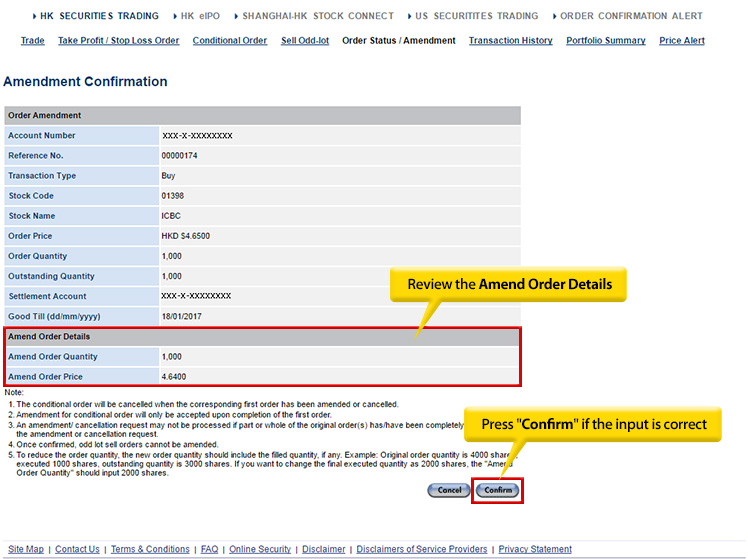This image is a screenshot from a securities exchange website with a white background. At the very top, there is a navigation bar featuring multiple tabs: HK Securities Trading, HKEIPO, Shanghai HK Stock Connect, U.S. Securities Trading, Order Confirmation Alert, among others, including options for trade management such as Take Profit/Stop Loss Order, Conditional Order, LODLOT, Order Status/Amendment, Transaction History, Portfolio Summary, Price Alert, and Amendment Confirmation.

The focal point of the image is a gray box titled "Order Amendment." Within this box, the following details are displayed: 

- **Account Number:** XXXXXXXXXX
- **Reference Number:** 00000174
- **Transaction Type:** Buy
- **Stock Code:** 01398
- **Stock Name:** ICBC
- **Order Price:** AHKD 4500
- **Order Quantity:** 1.000
- **Outstanding Quantity:** 1.000
- **Settlement Account:** XXXXXXXXXX
- **Good Till:** 18/01/2017

There is a prominent red-bordered box containing a yellow speech bubble that reads, "Review the Amend Order Details." The Amend Order details show:

- **Amend Order Quantity:** 1,000
- **Amend Order Price:** 4.64000

In the bottom right corner of the gray box is a red-bordered Confirm button, accompanied by another yellow box saying, "Press Confirm if the input is correct."